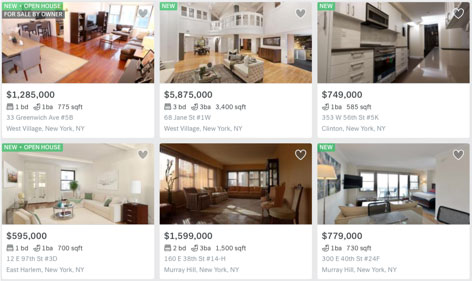The image is a screenshot of a real estate listing webpage featuring six properties. Each property is represented by a photograph and detailed information. 

1. **Upper Left**: The photo showcases a combined dining and living space designated as "New Open House" on a green background and "For Sale by Owner" on a black background. The property is listed at $1,285,000 and includes 1 bedroom, 1 bathroom, and 775 square feet. It is located at 33 Greenwich Avenue, Unit 58, West Village, New York, NY.

2. **Upper Middle**: This listing features an image of a living area with a balcony. It is located in West Village, New York, NY.

3. **Upper Right**: The photograph shows a galley-type kitchen. This property is situated in Clinton, New York.

4. **Bottom Left**: The image depicts a living room. The property is in East Harlem, New York, NY.

5. **Bottom Middle**: This listing displays a living room in Murray Hill, New York, NY.

6. **Bottom Right**: The photograph is slightly blurry and appears to show a living room in the background with a dinette in the foreground. This property is located in Murray Hill, New York, NY.